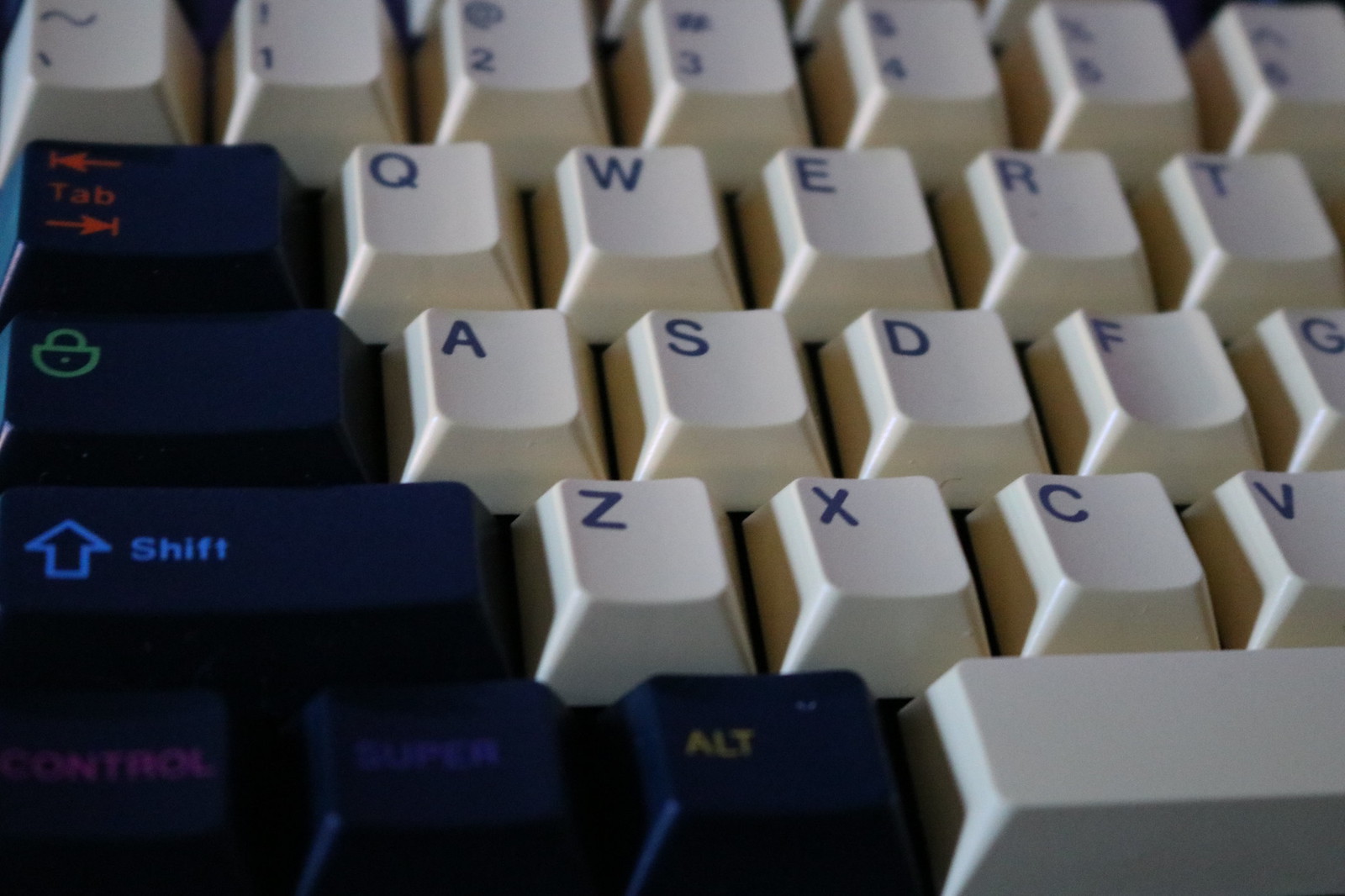This detailed close-up color photograph showcases a slightly dated computer keyboard, focusing on a few rows of keys. Most of the keys are white or beige with black lettering, including the number row from 1 to 6, though the numbers 4 through 6 are slightly out of focus. The alphabetic keys visible are QWERT in the top row, ASDFG in the second row, and ZXCV in the third row, along with a partial view of the spacebar, which is also white. 

On the left side, several black keys contrast with the predominately white/beige keys. These include a TAB key with red lettering, a shift key denoted by a blue up arrow, and a LOCK key featuring a green lock symbol. Additionally, there’s a black key labeled SUPER, a black CTRL key with pink lettering, and an ALT key with yellow-red coloring. Each key's function is clearly indicated, either by symbols or capitalized text, adding to the keyboard’s distinctive and slightly retro aesthetic.